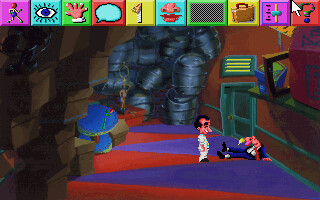This detailed screenshot from a vintage, 90s-style video game depicts a colorful and intriguing scene. Dominating the foreground are two human figures: one in a white outfit with black hair and another in a purple and black suit with a red tie, resembling a character in games such as Leisure Suit Larry. The man in the suit, characterized by his cartoonish large nose and smile, appears to be observing the other figure intently. They are situated in a room with a purple and red patterned carpet, wooden barrels on the right, and a pile of brown boxes on the left. The room's brown walls feature a green doorway and a vent, giving a sense of an old warehouse or storeroom.

Above the main scene runs a horizontal bar filled with various multicolored icons, each encased in squares of pink, blue, green, red, and yellow. These icons symbolizing different actions or tools include a running figure, an eyeball, a hand, a speech bubble, a zipper, a nose and mouth, a chessboard, a suitcase, a volume dial, and finally, a question mark with a hovering white computer mouse arrow. This collection of icons enhances the sense of the game's interactive and mysterious nature, further evidenced by the presence of a character lying on the ground and the overall detailed depiction of the vintage visual style.